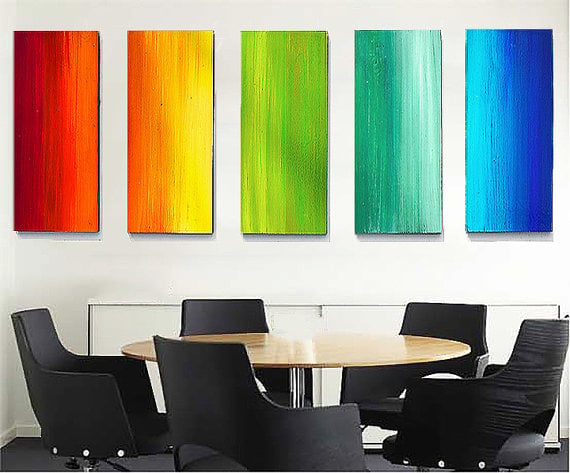This photograph captures a modern office conference room characterized by its clean, white walls adorned with five abstract paintings. Each artwork features vibrant, vertical gradients that blend seamlessly into one another, creating a spectrum effect from left to right. The sequence of colors transitions from red and orange in the first painting, to orange and yellow in the second, then yellow into green with slight red accents in the third, followed by teal and blue in the fourth, and finally light blue transitioning into dark blue in the fifth. 

Below the paintings, a round table with a wooden surface and a chrome, one-legged stand takes center stage. Surrounding the table are five swivel chairs with dark grey or black cushions and backrests, which add to the room's professional decor. A reflective, mirror-like surface is visible behind the chairs at the bottom of the image, enhancing the room's spacious and open feel. The overall style of the room is contemporary office decor, designed for both functionality and aesthetic appeal.